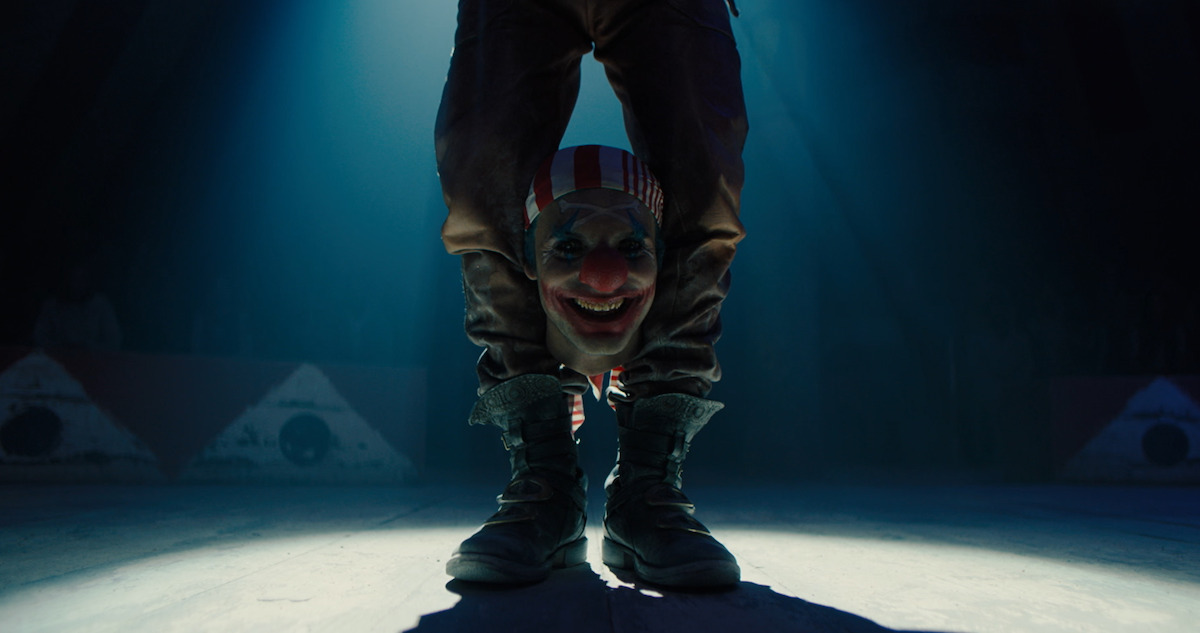The image is unsettling and surreal, featuring a pair of long legs clad in yellow pants and boots, captured from just above the knees down to the feet, standing under a spotlight. Positioned between these legs is a disembodied clown's head, evoking a sense of eerie peculiarity. The clown's face, reminiscent of the Joker, is adorned with heavy makeup including a large red smile and a red clown nose. Atop the head sits a bandana or a striped hat. The background is dark, with blurred, pyramidal white structures faintly visible, adding to the overall creepiness of the scene. The stark spotlight isolates the bodiless clown's head and the mysterious legs, heightening the bizarre atmosphere of the photo.